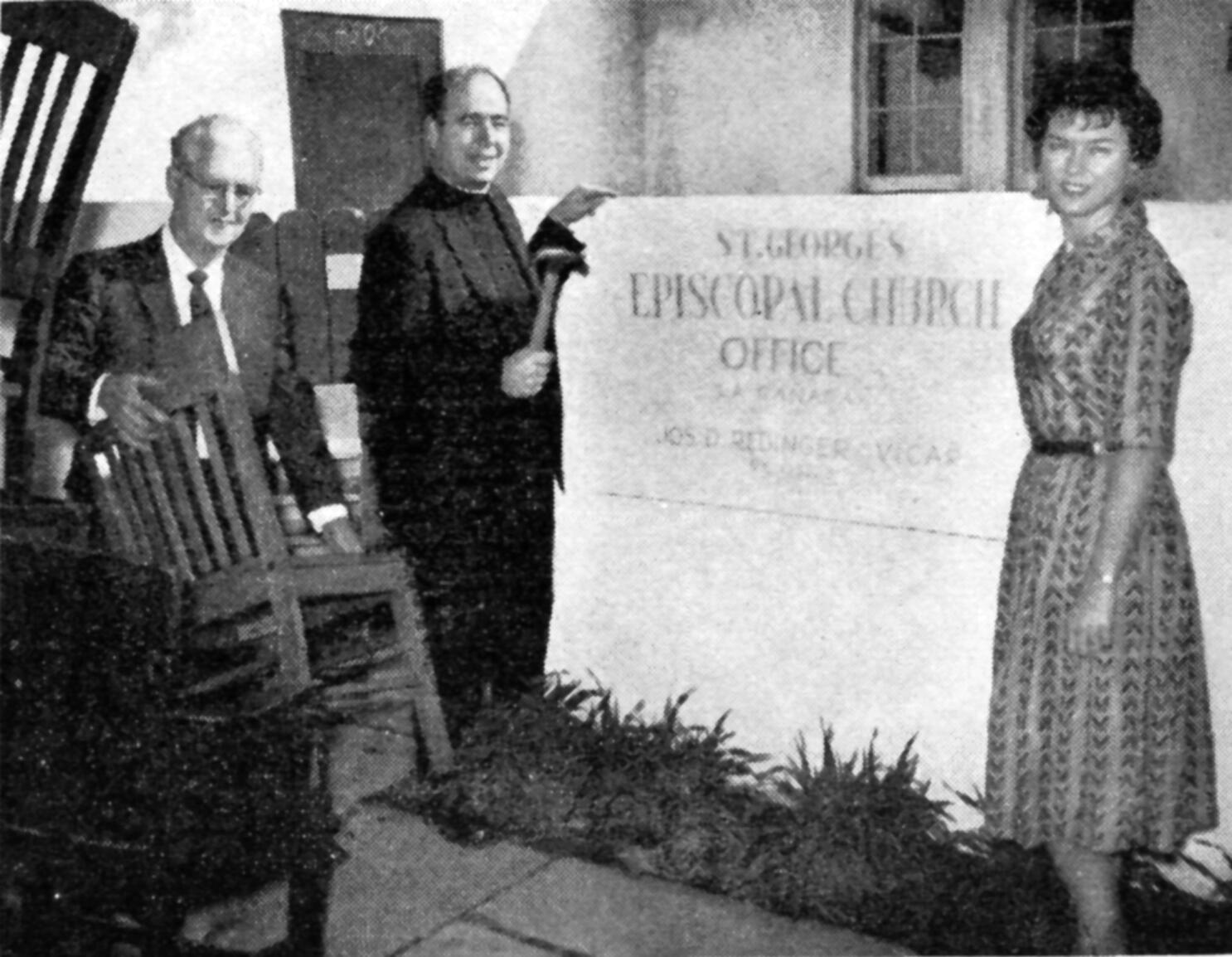This black-and-white photograph, taken a few years ago, features a staged scene in front of a sign for "St. George's Episcopal Church Office." The sign, attached to a white courtyard wall with partially obscured text underneath, indicates the setting. On the left side of the image, a man dressed in traditional Episcopal clerical attire, complete with a black suit and clerical collar, holds a hammer and gestures towards the sign. To his left stands another man in a regular black suit, carrying a chair. On the far right, a woman in a flower-patterned shirtwaist dress with elbow-length sleeves and a belted waist poses. Her short hair complements her vintage look. The group stands in front of what appears to be a courtyard, with the church building visible in the background. Despite the cohesion in their actions and expressions, there’s an unnatural quality to their arrangement, making the scene appear as if it were photoshopped, especially since the priest seems disproportionately close to the sign and the grass partially obscures their feet.